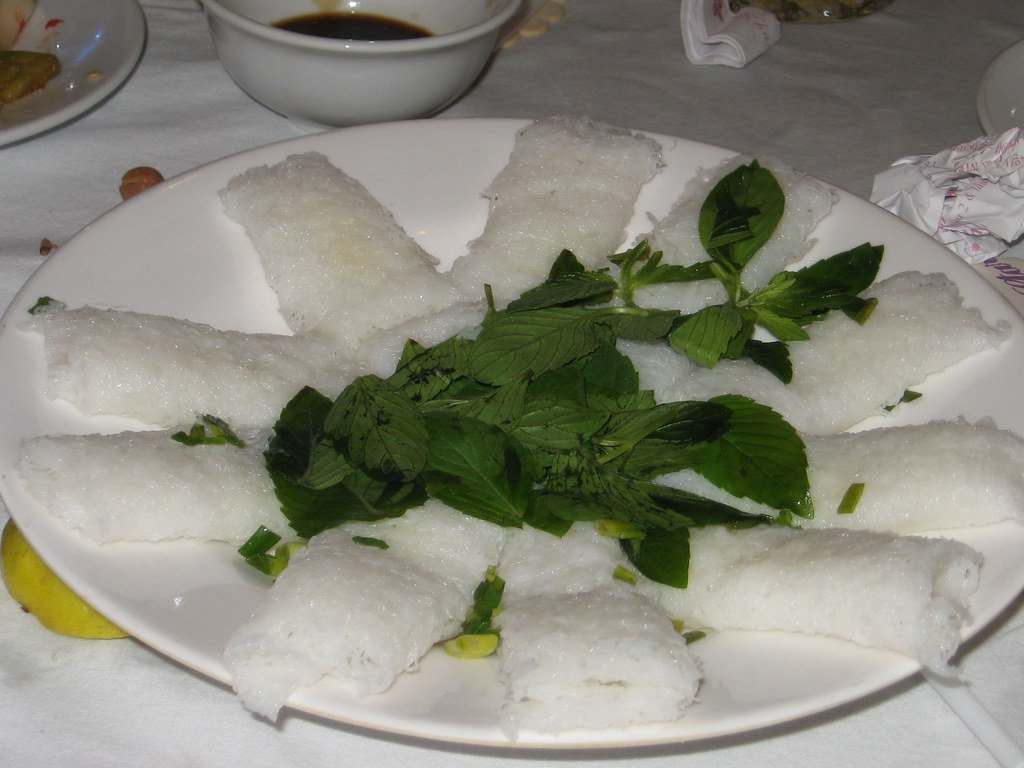In this close-up image, a distinct Japanese dish takes center stage. The focal point is a white plate brimming with meticulously packed white rice rolls, arranged in a star-like formation. Strategically placed around and on top of the rice are muddled green herbs, possibly mint or basil, suggesting a thoughtful preparation to extract maximum flavor. A hint of yellow oil drizzled on the rice adds visual appeal and flavor. The plate is supported or accompanied by a yellowish object, possibly a lemon, visible peeking underneath its left edge.

Directly behind the main plate is a circular bowl containing a brownish-orange broth, though its specific contents are not clearly visible. To the left of this bowl sits another plate with remnants of food and streaks of sauce, indicating it has been partially consumed. A folded piece of paper or napkin is seen in the background to the right, atop a white tablecloth that provides a clean, crisp backdrop. Scattered crumbs around the main plate enhance the impression of an authentic culinary experience being captured mid-way.